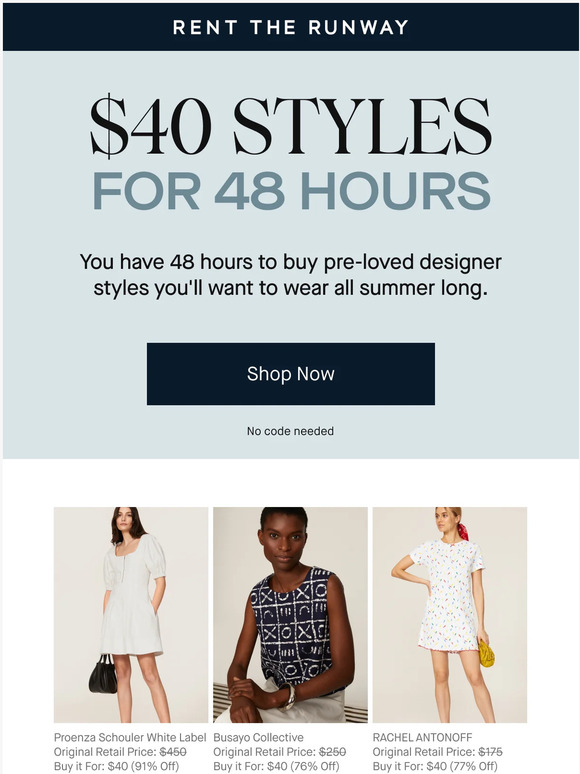The image features a promotional banner with a dark blue border at the top, displaying "RENT THE RUNWAY" in bold, white capital letters. Below this, a light blue background holds prominent black text reading "$40 STYLES." Underneath, gray text announces "for 48 hours," followed by black text explaining "you have 48 hours to buy pre-loved designer styles you will want to wear all summer long." A black rectangular box sits below with "SHOP NOW" written in white in the center, and "No code needed" stated underneath.

The bottom portion of the image showcases three thumbnails. The left and right thumbnails each depict a woman modeling nightgowns, while the middle thumbnail shows a person, possibly male or female, wearing a tank top with a tic-tac-toe pattern. Below the left image, text reads "Proenza Schouler White Label: Original Retail Price $450, Buy it for $40 (91% off)."